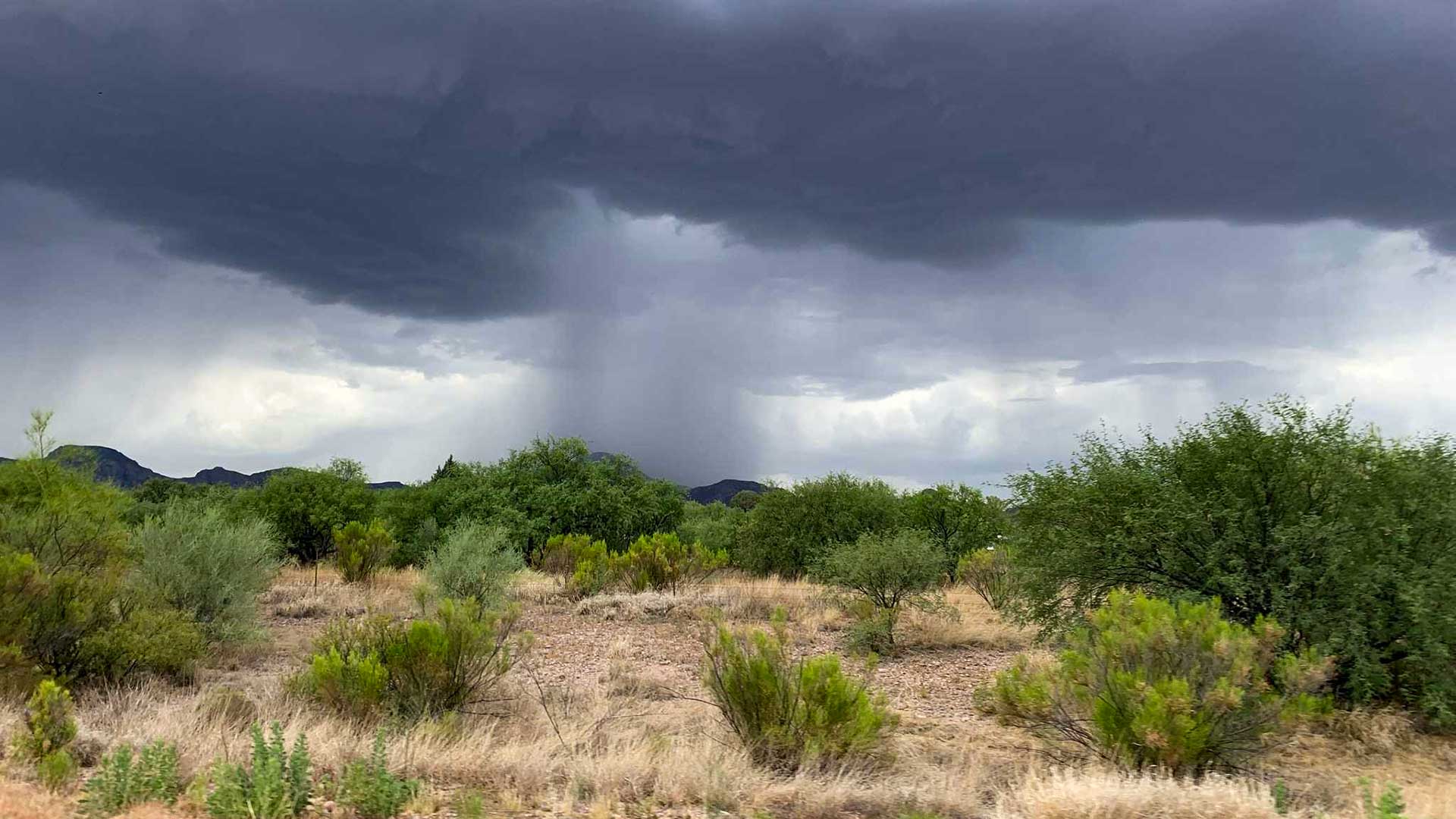A wide-angle distant shot captures a stark desert landscape in the foreground, where sparse, large green bushes and dry, long, khaki-colored grass dominate the scene. The terrain is barren, with randomly scattered shrubbery and patches of open, dusty earth. In the distance, low mountain peaks faintly outline the horizon. Dramatic contrasts paint the sky; dark gray, thick storm clouds loom overhead, interspersed with streaks of brighter white clouds hinting at sunlight piercing through their edges in the top left corner. The center of the image showcases a striking spectacle—a light gray wall of rain descending from the clouds, reaching the ground, while the foreground remains dry. This intense wall of rain, or rain shaft, vividly splits the image between the arid foreground and the storm-engulfed background, emphasizing the dramatic weather contrast in this desert terrain.